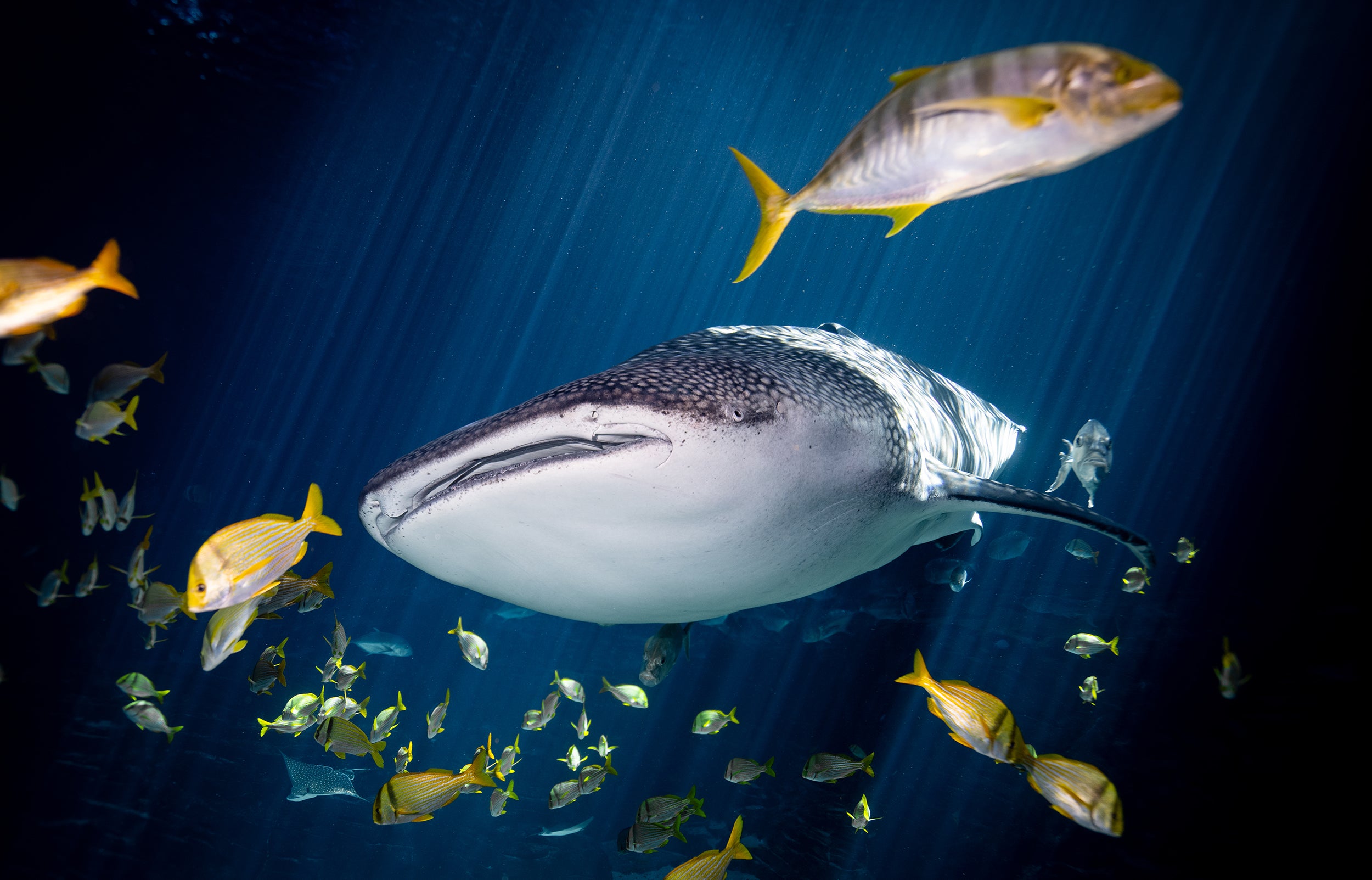The underwater scene appears as a highly detailed and artistic rendering, possibly created with AI technology. Dominating the center of the image is a majestic whale shark, its large, flat mouth and distinctive gray body dotted with white patterns clearly in view. The ocean backdrop is a deep, dark blue, almost black, with beams of light penetrating the water and illuminating the tops of the fish, casting a mystical glow on the marine tableau.

Surrounding the whale shark is a lively array of marine creatures. Starting from the top right and weaving around the giant shark, a school of various fish, primarily yellow in color and some with gray stripes, moves in unison. Among these, a larger fish, possibly a yellowfin tuna, hovers above the whale shark. Several smaller fish, identified by their tiny yellow fins, swim alongside and beneath the shark. 

Adding to the rich diversity of the scene, a spotted stingray glides gracefully beneath and to the left of the whale shark. Farther back, a manta ray can also be spotted, its broad wingspan creating a silhouette against the faint blue light. Some of the fish in the foreground appear slightly blurry, hinting at their swift movements or proximity to the camera, contributing to the lifelike quality of the scene. Overall, the image captures the serene yet vibrant underwater world with remarkable detail and artistic finesse.